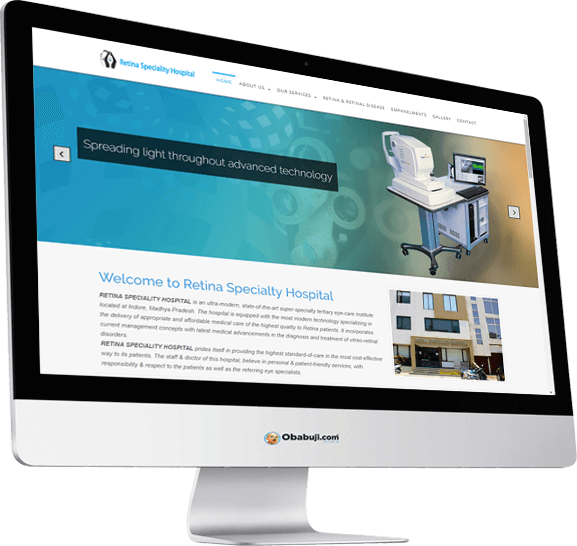A sleek flat-panel monitor, featuring a black bezel and a silver stand with a silver bar at the bottom below the bezel, displays the website for Retina Specialty Hospital. Dominating approximately one-third of the screen, a prominent graphic features a gradient background transitioning from blue to brown. The graphic showcases a sophisticated white eye-examination machine mounted on a roller table, complete with a head strap and chin rest for patient support, as well as an adjacent computer for data analysis. The displayed text reads, "Spreading light through advanced technology." Below the graphic, in the lower right corner, there is an image of the hospital accompanied by the text "Welcome to Retina Specialty Hospital," which becomes increasingly small and difficult to read. Additionally, seemingly added post-capture, the monitor displays an incongruous round circle with a blue rim and an image of a baby's face, alongside the name "Obabuji.com." The perspective of this addition appears misaligned with the monitor's frame, suggesting it was superimposed later.